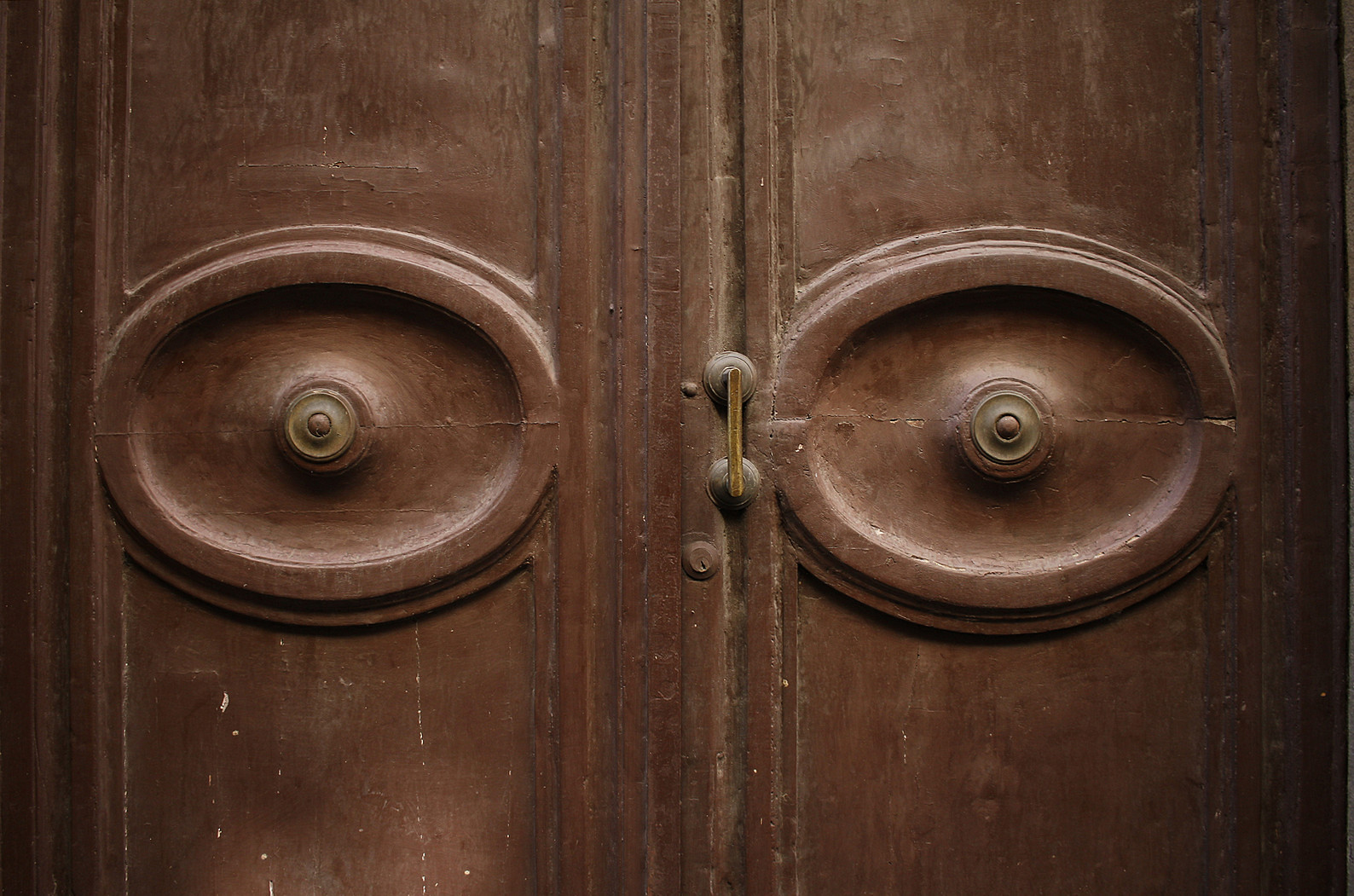This landscape-oriented photograph captures a pair of antique wooden doors reminiscent of those found on old European buildings. The doors, rich with brown hues and textured surfaces, feature a symmetrical design divided by a central line, with each door opening left and right. Both panels display an ornate, oval-shaped carving at their centers, giving the impression of eyes when viewed together. Within each oval is a decorative round metal plate composed of concentric circles, with the innermost circle in a dark green color. The right door is equipped with a gold handle mounted on two brass plates, and a small metal keyhole below it. The intricate and vintage design elements of these doors not only enhance their aesthetic appeal but also evoke a sense of historical elegance.